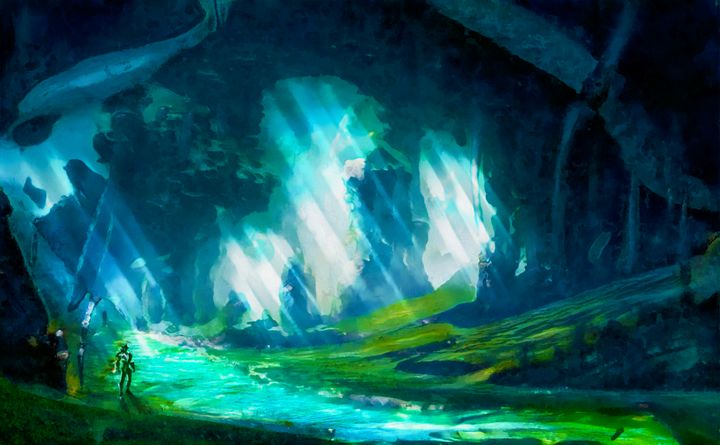This meticulously detailed watercolor painting portrays an ethereal underwater cave scene primarily rendered in deep and light shades of blue, reflecting the submerged nature. At the top, the cave structure is composed of deep navy tones with multiple openings, through which sunlight streams in, casting Jacob's ladders in light blue and white hues that add a mystical glow. Descending from this lit area, a grassy, sloped hill transitions into a small river channel, subtly flowing from the back left to the bottom right. The river’s water contrasts in a slightly different blue, enhancing the serene ambiance. In the bottom left corner, a figure dressed in green clothing with white accents stands on the bank, gazing towards the water. Near this figure, a sea serpent can be seen gracefully swimming above, adding an element of fantasy. The scene is impressionistic with deliberate stretches and diffusions, lending it an otherworldly, poetic feel. Additionally, hints of more figures are discernible behind the primary one, leaning against a rock structure, further enriching the narrative depth of this underwater spectacle.